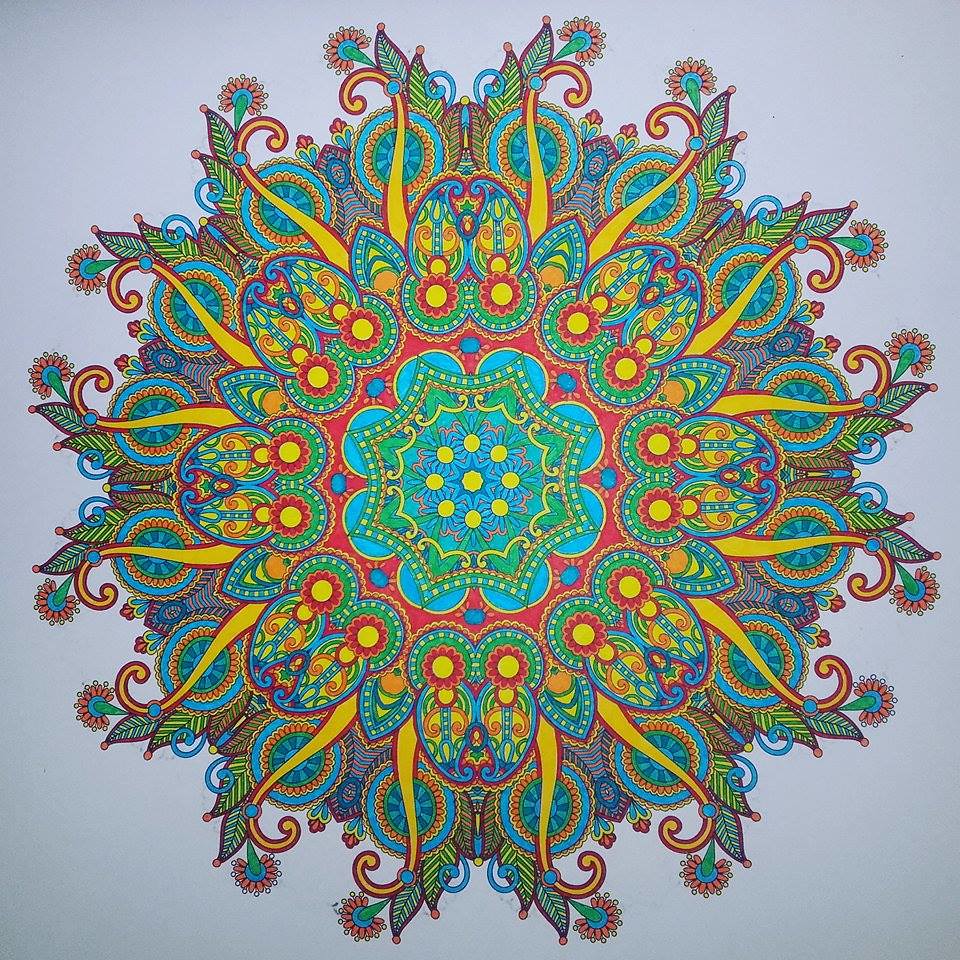This digital artwork features an intricate, kaleidoscopic design that captivates the viewer with its vibrant colors and symmetrical patterns. At the base of the composition, a striking yellow orb is encased within a geometric blue star. Each tip of this star is adorned with a yellow orb, connected by elaborate blue floral motifs. These floral designs gracefully transition into yellow, curved bands that seamlessly connect to an undulating green scalloped band, creating a rhythmic visual flow. Within the spaces between the scalloped edges, blue half-circles radiate outward, adorned with accents of yellow and red, adding depth and complexity to the overall piece. The meticulous detailing and harmonious color palette make this artwork a mesmerizing visual experience.